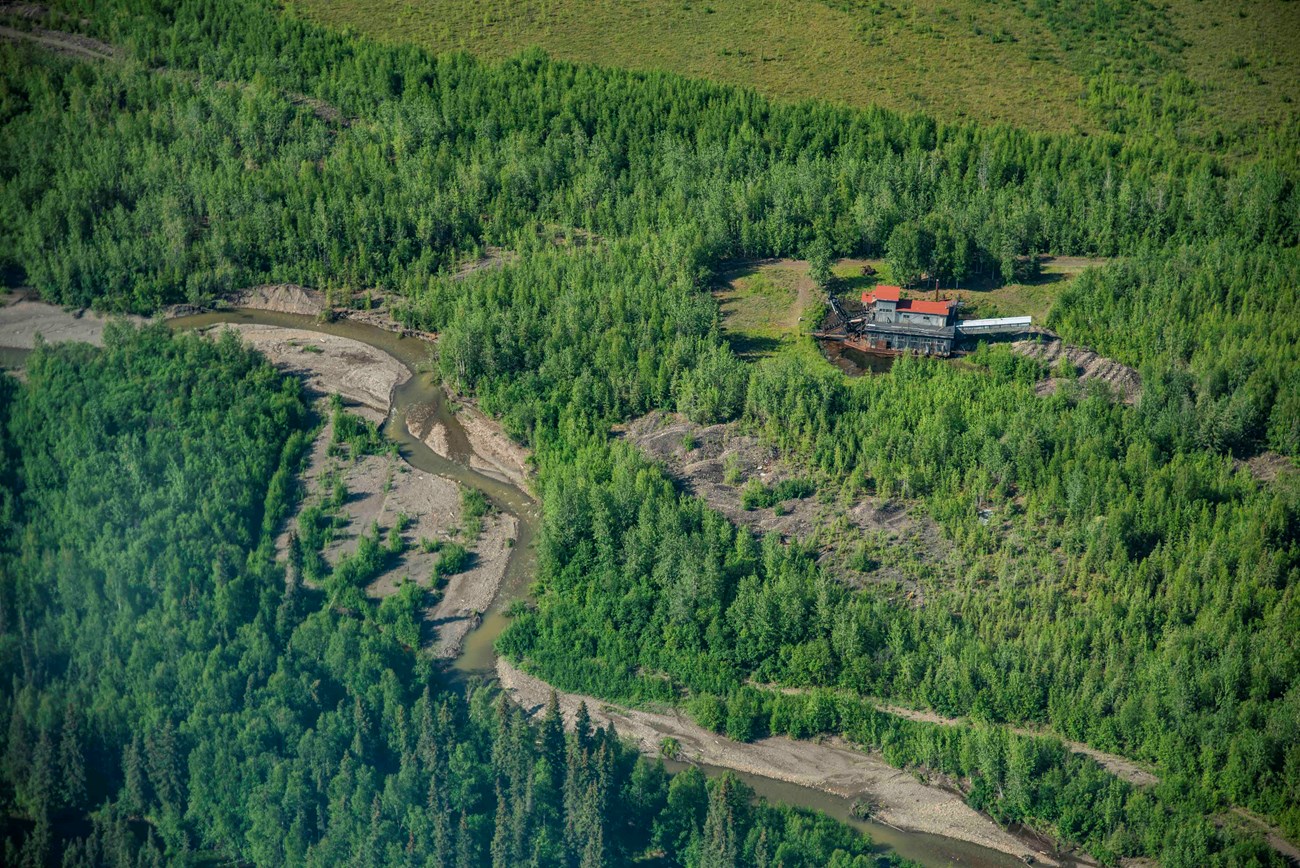This aerial daytime photograph beautifully captures a lush, green landscape dominated by an expansive forest of evergreen trees. In the center of the image, a winding, thin river gracefully curves its way through the dense greenery, adding a dynamic flow to the scene. Towards the far right, there's an intriguing structure resembling an old dredging boat, used historically for gold extraction, resting in an almost empty body of water. This boat-like structure, which appears to have been abandoned for years, is reminiscent of a houseboat with distinctive arms for dredging.

In another part of the image, nestled amidst the green expanse, stands a lone, two-story house with a striking red roof and blue walls. Adjacent to it is a possible bridge, seemingly constructed to cope with potential flooding from the nearby river. The land slopes gently upwards towards a hilltop, covered sparsely with grass, and offering little resistance to heavy rains or floods. The absence of neighboring houses accentuates the solitude and seclusion of this picturesque abode, surrounded by the serene beauty of vibrant, lush trees.